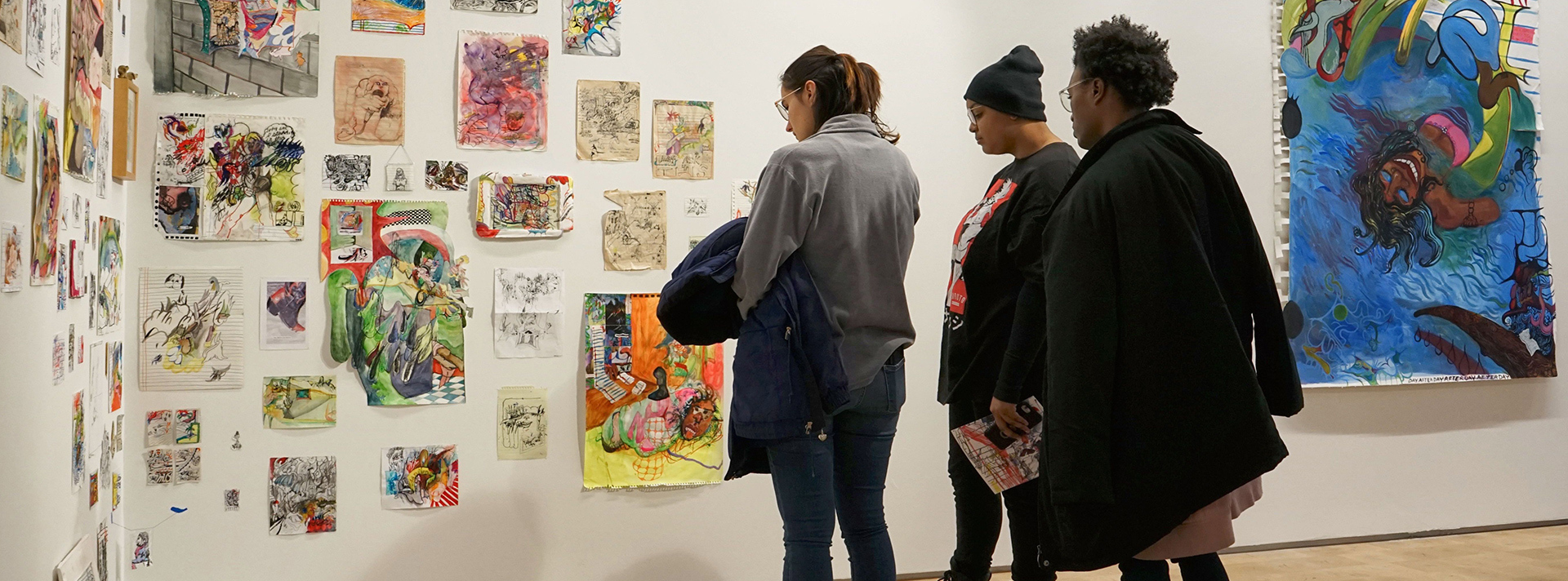The image depicts three women examining an array of colorful artwork on an off-white wall in what appears to be a gallery or classroom setting. The wall is adorned with numerous pastel and vivid colored pieces of unframed art, affixed with tape or thumbtacks, reminiscent of a parent night at a child’s school. To the right of the group, a large canvas in shades of blue, rose, green, and black hangs prominently. The woman at the front has auburn hair, wears a gray shirt and jeans, and carries a dark coat under her left arm. Behind her stands a woman in a dark shirt with a logo, wearing a knit stocking cap, holding a piece of paper or magazine and a phone in her left hand. The third woman, partially visible with a pink dress peeking from beneath a black jacket, completes the trio. The artwork, mainly abstract, varies in size from smaller than a standard sheet of paper to as large as an average poster. Notably, the large painting on the right appears to depict an African American girl against a blue sea backdrop, her face and body oriented upwards.